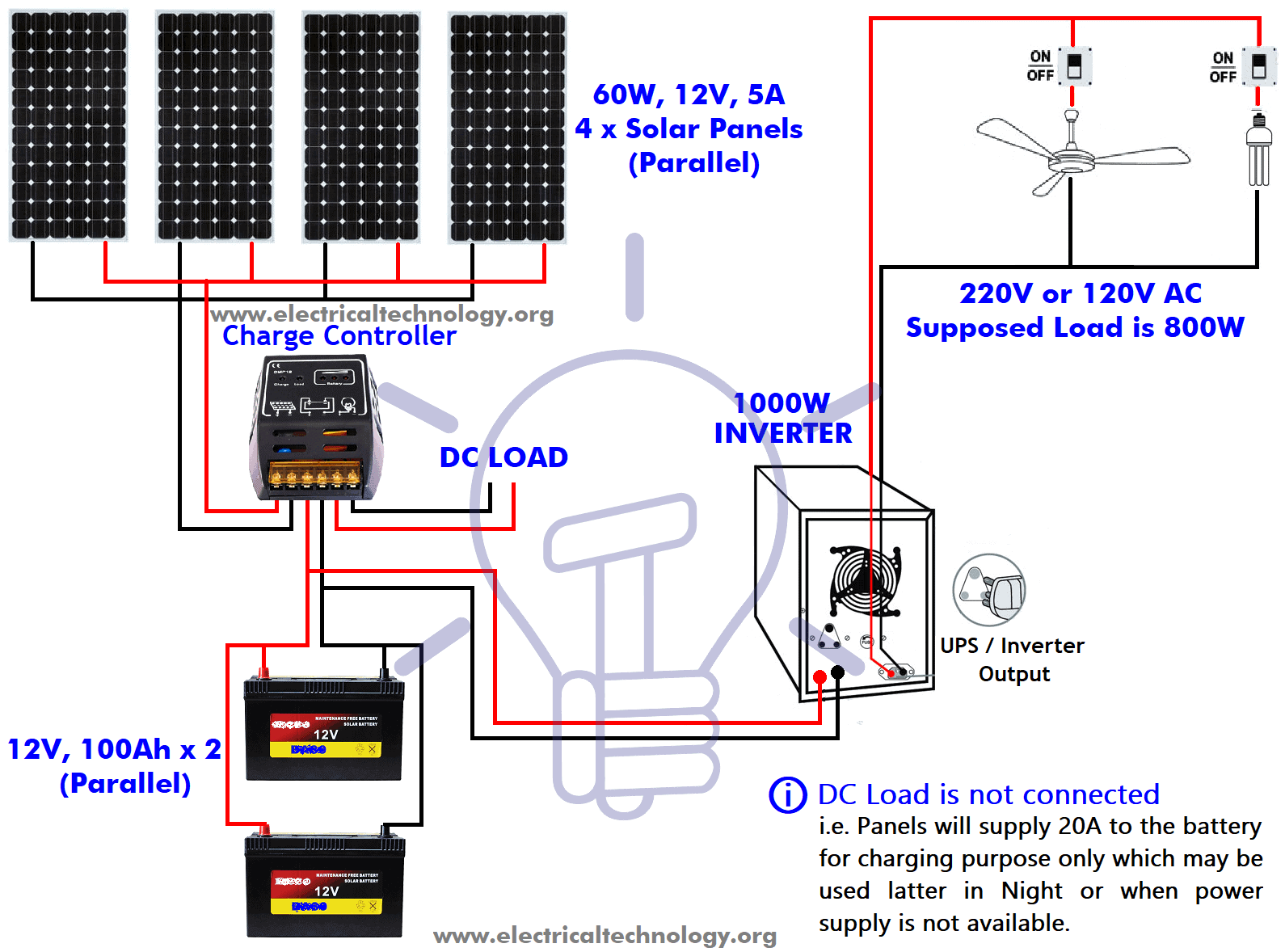This image is a detailed schematic diagram illustrating the connection and functioning of a solar power system. Against a solid white background, in the upper left corner, there are four vertically aligned black rectangles with small white dots labeled as solar panels. Each panel is specified as 60W, 12V, and 5A, and are connected in parallel. Red and black lines descend from these panels connecting them to various components of the system.

To the right of these panels, blue text labels them again as 60W, 12V, 5A, four times in parallel. Directly below, a blue-labeled "charge controller" is represented by a black rectangular box with gold knobs on its edges. Further connections in red and black lines lead from the charge controller to a pair of 12V, 100Ah batteries, also connected in parallel.

On the bottom right, another red and black connection moves towards a "1000W inverter” depicted as a box with a central fan. Additionally, in the upper right portion of the diagram, a ceiling fan with three blades, labeled with an on/off switch, is connected to the system. It is specified to operate at either 220V or 120VAC with a supposed load of 800 watts.

Notably, the DC load is specified as “not connected” and the schematic suggests that the panels will supply 20A to the batteries for charging purposes, which can be utilized later when the power supply is unavailable. At the bottom of the diagram, the website "www.electricaltechnology" is noted, potentially for further information.